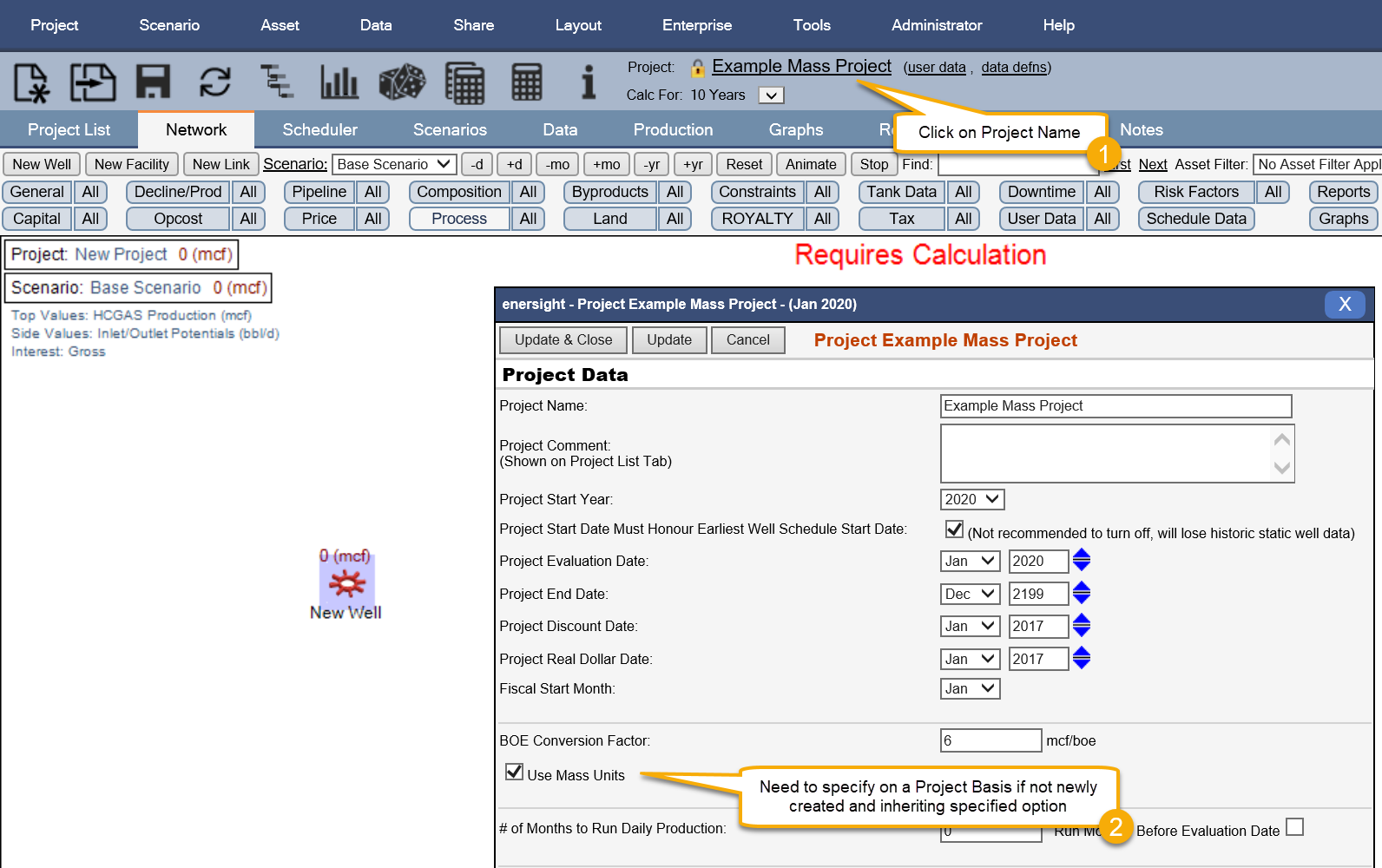Here’s the refined and detailed caption for the picture described:

The image showcases a software interface, presumably for project management or data analysis. The interface features a predominantly white background with three distinct banners at the top:

1. The topmost banner is dark blue with white font, displaying various categories such as Project, Scenario, Asset, Data, Share, Layout, Enterprise, Tools, Administrator, and Help.
2. Below it, a bluish-gray banner contains buttons for actions such as Select, Copy, Save, and Refresh, alongside Calculator and Information icons.
3. The third banner, a darker bluish-gray shade, holds the project name, which includes the text "C-A-L-C for 10 years."

Underneath these banners, there are several tabs for different functionalities: Project List, Network, Scheduler, Scenarios, Data, Production, and Graphs. A yellow-outlined speech bubble with black font on a white background instructs, "Click on the project name," marked with a yellow bubble containing the number 1.

Further elements on the interface include various buttons and filters. The main section of the screen highlights a message in red font stating "Requires calculation" and another labeled box titled "Project Example Mass Project." This box contains specific project data and is accompanied by a second yellow-outlined speech bubble with the instruction, "Need to specify on a project basis if not newly created and inheriting specified option," marked with a number 2.